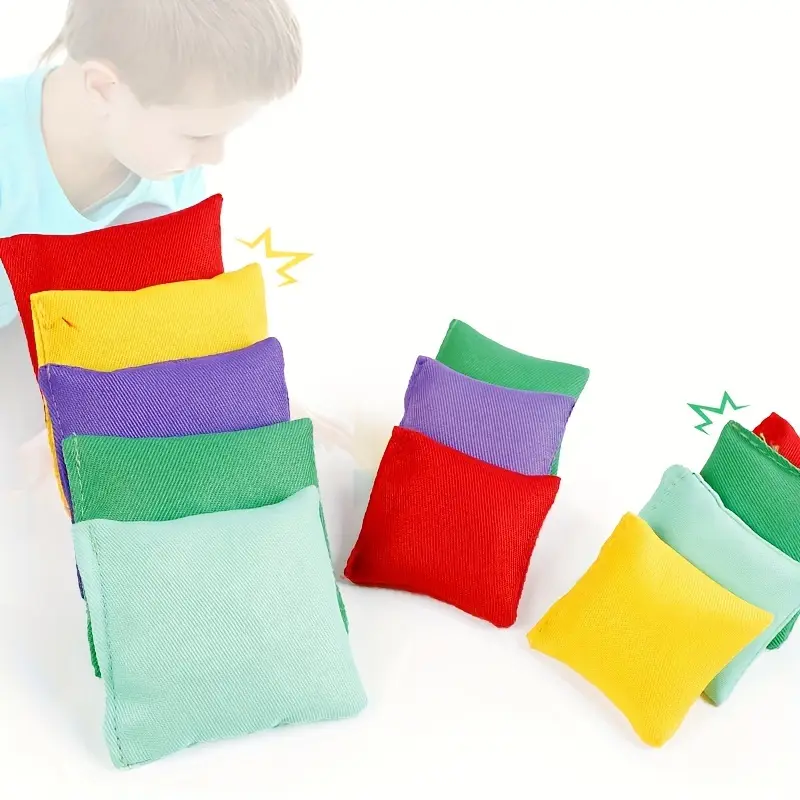This product photo showcases an array of square cornhole sacks in a variety of vibrant colors set against a pristine white background. Arranged meticulously, the left side features five larger sacks in the order of red, yellow, purple, green, and light green. The right side displays rows of smaller sacks, colored in red, yellow, purple, green, light blue, and a mint hue. These sacks, reminiscent of small, fluffy pillows, have yellow and green zigzag patterns adorning their sides, adding a decorative touch. To the top left, there is an ethereal image of a boy with short brown hair and a distinctive rat tail haircut, wearing a blue shirt. This ghostly overlay adds an intriguing, semi-transparent element to the otherwise professional, well-lit product photograph.